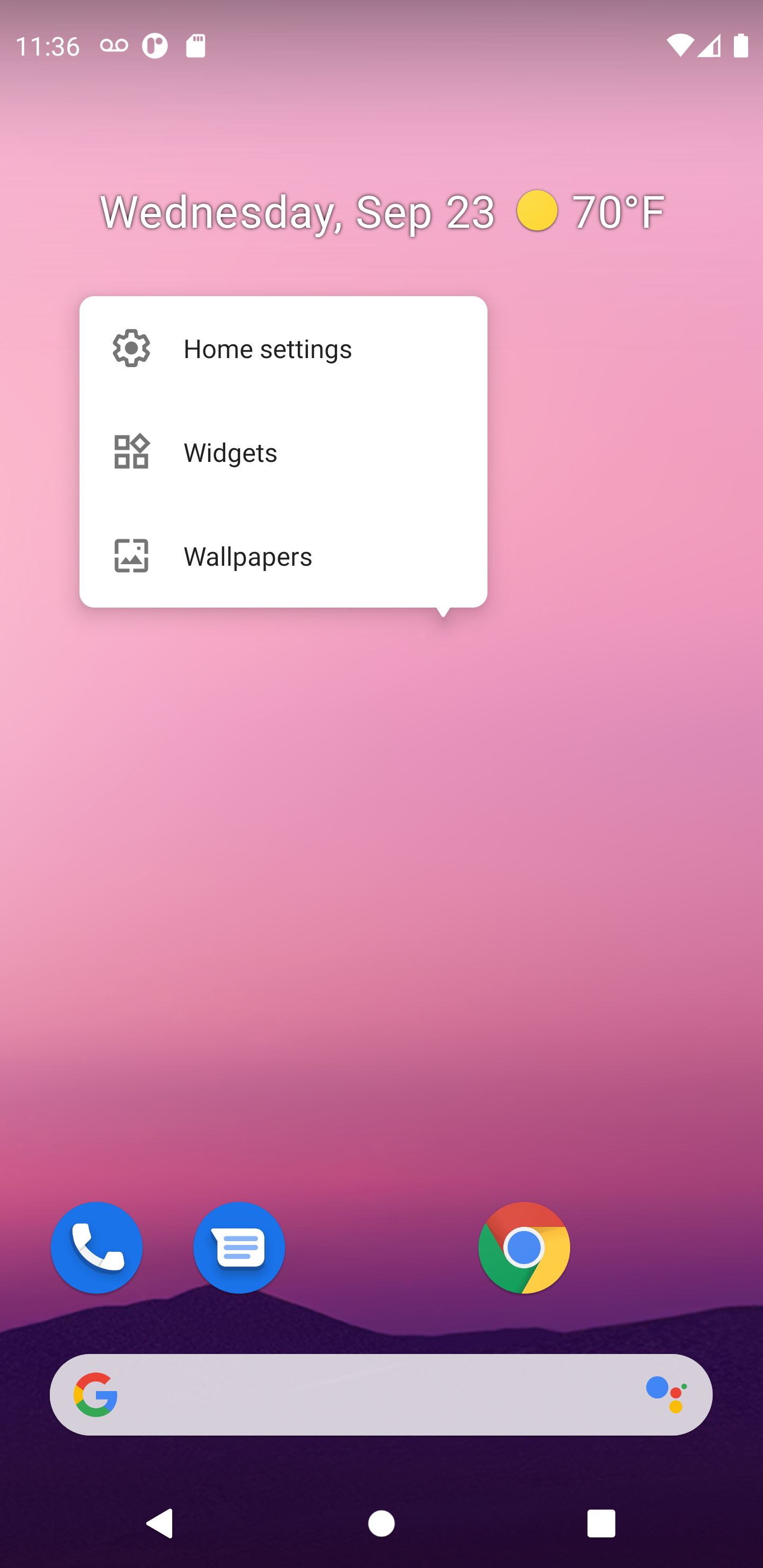The screenshot captures the vibrant and colorful home screen of a smartphone. The background features a gradient that transitions from a pastel pink at the top to a rich burgundy or lavender at the bottom, resembling a serene mountaintop or mountain range. At the top of the screen, the time is displayed as 11:36, accompanied by a record icon and two other unidentified icons. On the far right, there are icons for Wi-Fi and battery status.

Below the time, in the center, the date is shown as "Wednesday, September 23rd," with a sunny weather icon indicating a temperature of 70 degrees Fahrenheit. Directly below this, there is a white box containing a settings wheel icon labeled "Home settings," a widgets icon labeled "Widgets," and a wallpaper icon labeled "Wallpapers."

Further down, there is a row of app icons, including the phone app, a document app icon, and the Google logo. Below this, a search box features the Google logo, followed by the Google colored circles: a blue circle, a red circle, an orange circle, and a lighter blue circle.

At the very bottom of the screen, navigation buttons are displayed: a left-facing arrow for back, a circle for the home button, and a square for recent apps. The overall layout is clean, with a clear structure and an aesthetically pleasing color scheme.